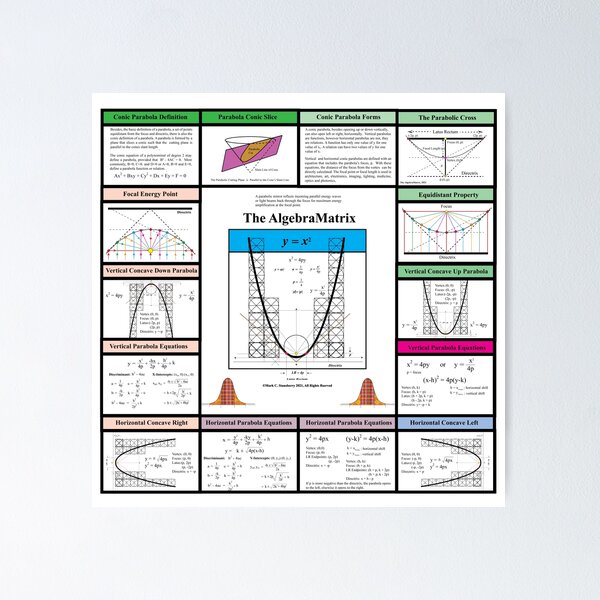This image is a detailed chart with various mathematical equations and explanations. The central and largest area, more of a rectangle shape, is labeled "The Algebra Matrix" and prominently displays the equation \( y = x^2 \) along with a corresponding diagram. Surrounding this central matrix, there are 14 smaller boxes. These smaller boxes contain different mathematical equations, graphs, and parabolic shapes, each with distinct bold headings in varying colors including green, blue, pink, and purple. Starting from the top, there are four blocks across, with four more blocks running down each side, minus the four at the top. At the bottom are two additional equations in the center. There are parabolas, horizontal concave shapes, and other geometrical and algebraic figures, each clearly marked and differentiated by their unique colorful headings.